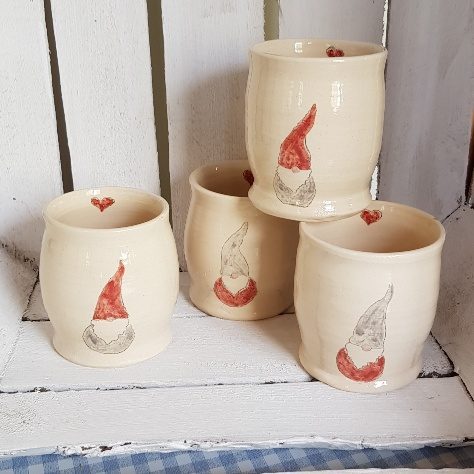This digital photograph captures a square-shaped image featuring four nearly cylindrical, cream-colored mugs adorned with illustrations of gnomes in red and grey. The mugs, handmade and handle-less, slightly curve at both the top and bottom, giving them a subtle hourglass shape. These mugs are arranged inside an open wooden container, painted white, with three mugs on the surface and the fourth balanced on top of two others. The container rests on a blue and white checkered tablecloth that partly peeks through at the bottom. The scene's colors include beige, red, grey, blue, and white, contributing to a charming and rustic aesthetic.